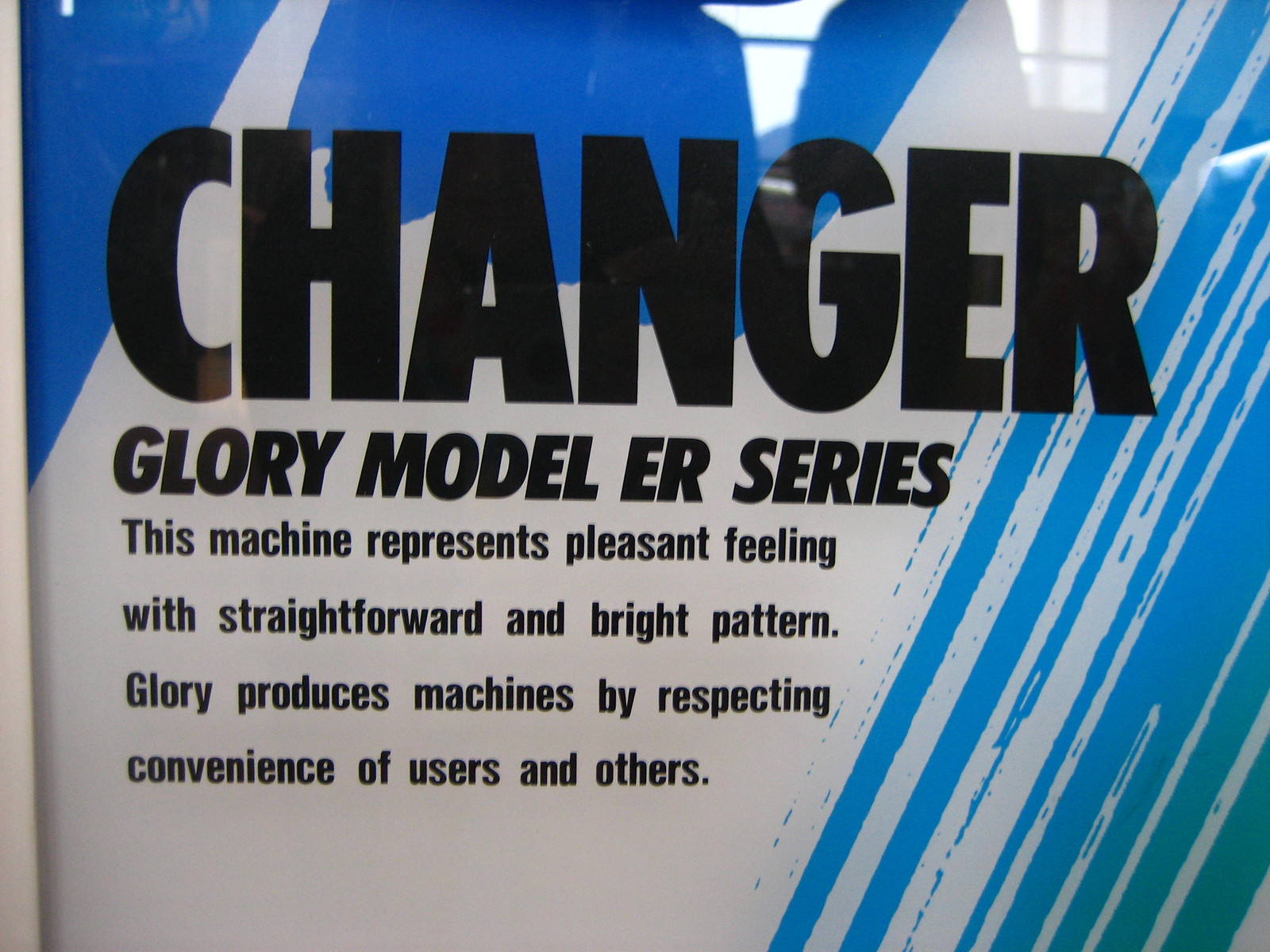The image is a close-up photograph of an advertisement for a machine, featuring text on what appears to be a metallic or glass surface. Dominating the top section of the ad is the word "CHANGER" in bold, black letters. Just below it, in a smaller font, it reads "Glory Model ER Series." The descriptive text beneath states, "This machine represents a pleasant feeling with a straightforward and bright pattern. Glory produces machines by respecting the convenience of users and others." The entire message is in English.

The advertisement's background has a combination of white and blue colors, including blue line patterns, particularly on the right side and around the edges. There's a noticeable reflection at the top, likely from a light source, indicating that the material could be glossy or behind glass. The text and patterns suggest a modern, sleek design, but the exact purpose of the machine remains unspecified. The overall impression is of a well-designed promotional piece emphasizing user convenience and aesthetic appeal.